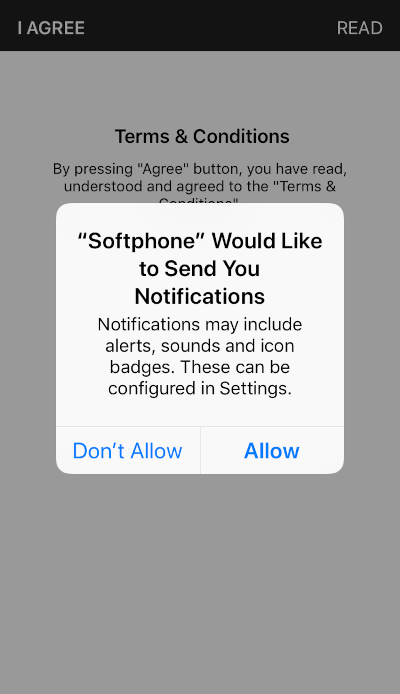In the image, a smartphone screen displays a permission notification prompt overlaying a grayed-out terms and conditions document. The permission request, encased in a white pop-up with rounded corners, originates from an application named "Soft Phone" (indicated in quotation marks). The header of the prompt asks, "Soft Phone would like to send you notifications," followed by a subtext that mentions these notifications may include alerts, sounds, and icon badges, all of which can be configured in the device's settings.

At the bottom of the pop-up, there are two response options in blue font: "Don't Allow" on the left and a bolder "Allow" on the right. Above, the navigation options "I Agree" on the left and "Read" on the right confirm the user's review and acceptance of the terms and conditions upon interaction. The screen lacks any additional interface indicators, such as time or battery status, focusing solely on the user’s interaction with the permissions and terms agreement. "Soft Phone" appears to be a software-based communication service, likely akin to Skype or other VoIP applications, facilitating voice and possibly video calls through internet protocols rather than traditional telecom networks.